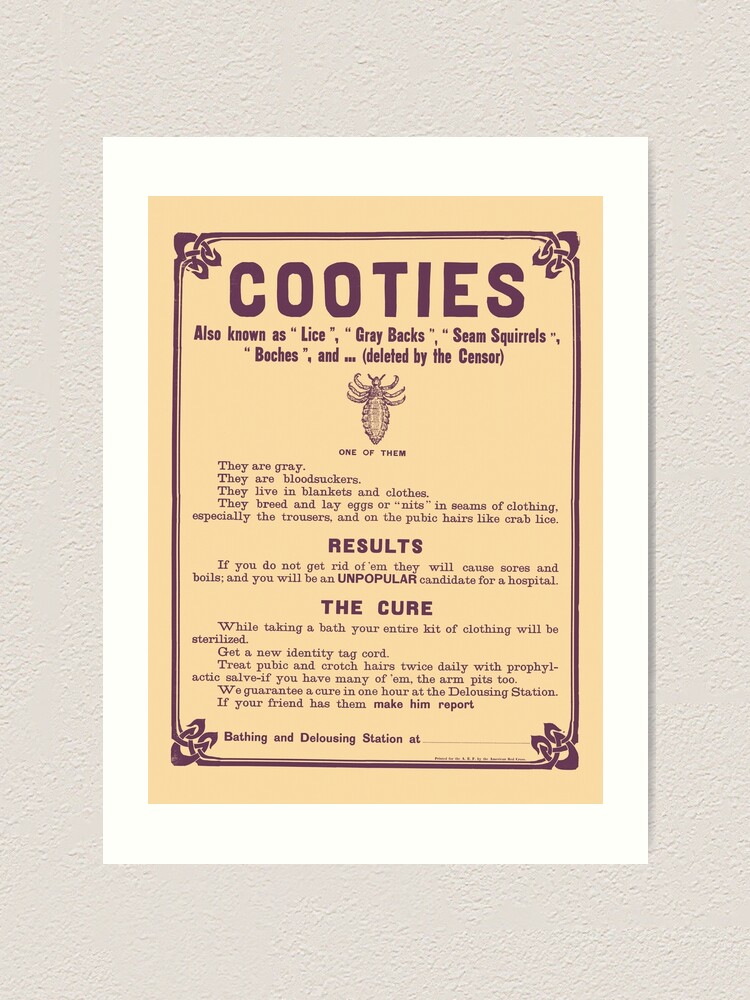The photograph depicts a white piece of paper hanging on a slightly eggshell-white wall, which has a light brownish-gray tinge. The paper is rectangular, about 5 to 6 inches high and 4 inches wide, and contains a flyer with instructional content about "Cooties," which is also spelled out at the top in large mauve print. The flyer describes cooties, also known as lice, graybacks, seam squirrels, moches, and one term that is noted as "deleted by censor." The background color of the flyer is a mix of yellow and sherbet orange, and it has a darker mauve border. 

The flyer includes a drawing of a louse, depicted as a spider-like creature with all its legs upfront, beneath which it reads, "one of them." The text follows: "They are gray, they are bloodsuckers, they live in blankets and clothes. They breed and lay eggs in the seams of clothing, especially in trousers and on pubic hairs like crab lice. Results: If you do not get rid of them, they will cause sores and boils, and you will be an unpopular candidate for a hospital," with the word "unpopular" emphasized in larger, bolder font.

The flyer also outlines a cure, stating: "While taking a bath, your entire kit of clothing will be sterilized. Get a new identity tag cord. Treat pubic and crotch hairs twice daily with prophylactic salve, and if infested heavily, treat armpits too. We guarantee a cure in one hour at the delousing station. If your friend has them, make him report. Bathing and delousing station at ______," with a blank line left for location details.